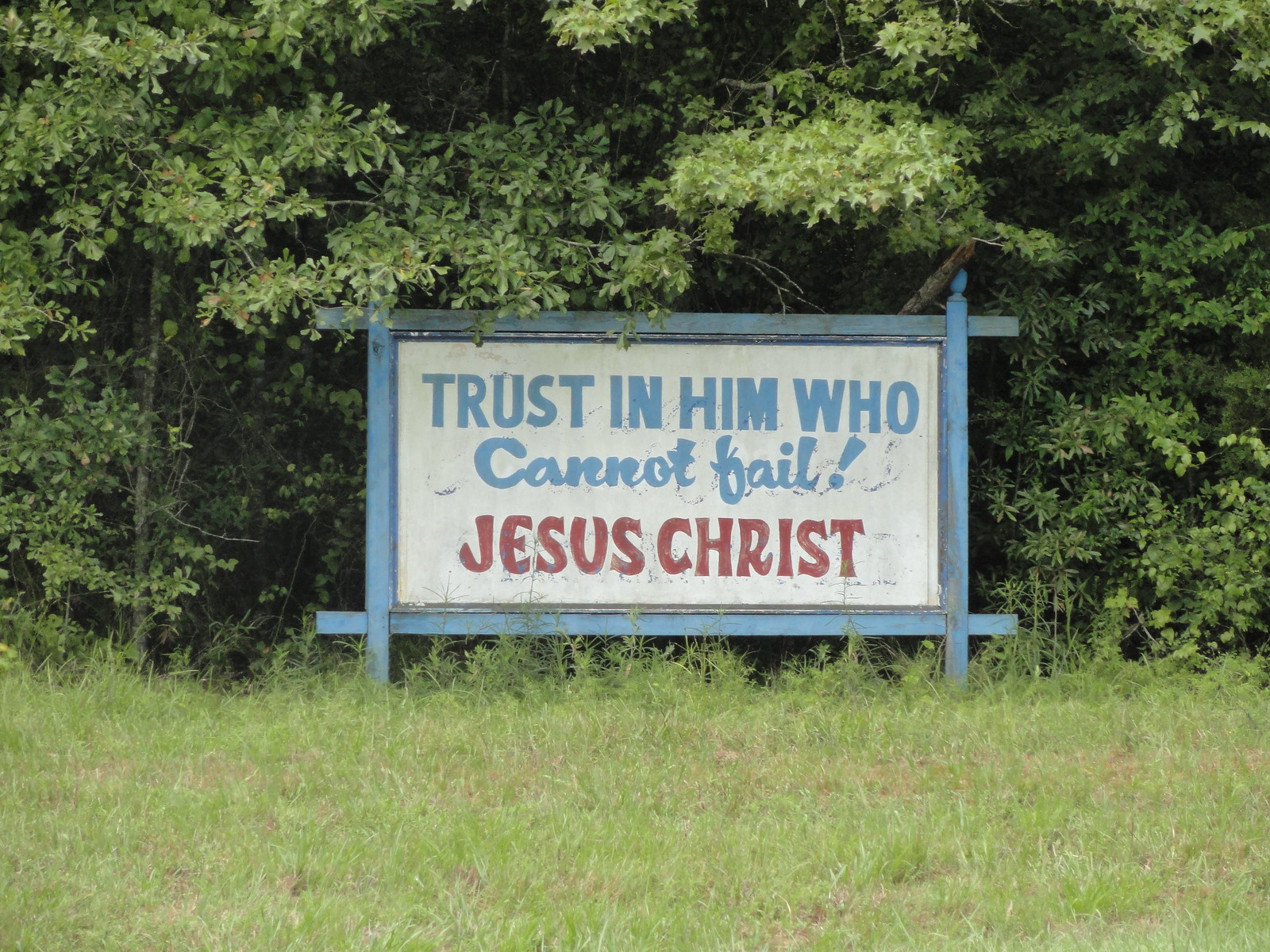A roadside sign is prominently displayed, measuring approximately eight feet by six feet. The structure is supported by blue posts that intersect at the corners, resembling the design of a picket fence. Within this frame, a white sign features bold blue lettering in all caps, which reads "TRUST IN HIM WHO". The message then transitions to elegant cursive, still in blue but not in all caps, stating "CANNOT FAIL!" The final part of the message is in bold red print, all caps, declaring "JESUS CHRIST." The sign stands in an open field, with a dense forest of trees providing a picturesque backdrop.